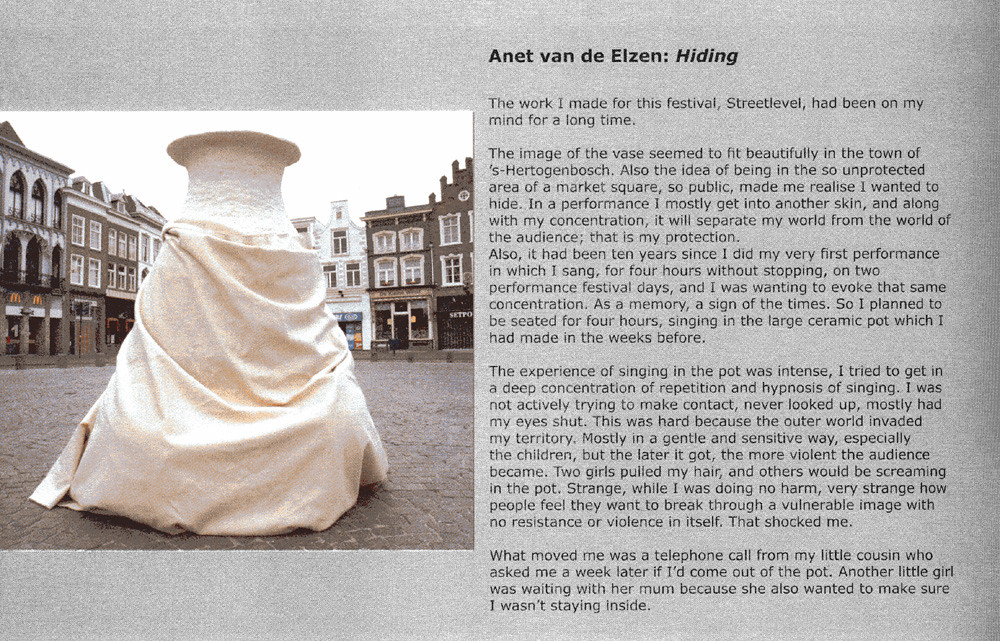This image appears to be a scan or photograph of a public information sign against a rough, grey background, reminiscent of old-fashioned TV static. On the left side, there is a depiction of a white draped sculpture, potentially a large ceramic vase, set in a cobblestone square surrounded by white, brown, and stone buildings with numerous windows. This scene is likely in the town of 's-Hertogenbosch.

At the top of the sign, bold black text reads "Annette van de Elzen," followed by the italicized word "Hiding." The accompanying text provides an in-depth description of the performance. It details how the artist created the work for a festival and chose the open, unprotected setting of a market square to evoke vulnerability and hiding. Annette van de Elzen reflects on her first performance a decade earlier, seeking to recreate the intense concentration from singing for four hours without stopping.

For this recent piece, she planned to sit and sing within the large ceramic pot she created, aiming to enter a state of deep concentration and repetitive hypnosis. Despite her efforts to disengage, never looking up and mostly keeping her eyes shut, the outer world's presence was unavoidable. Early on, children interacted gently, but as time passed, audience behavior turned violent, with two girls pulling her hair and others shouting into the pot. This aggressive response to her passive, vulnerable image shocked her deeply. A week later, a touching moment occurred when her little cousin called to ask if she had come out of the pot, and another young girl and her mother waited to ensure she wasn't still inside.

The detailed narrative, juxtaposed with the visual of the draped ceramic vase, vividly captures the artist's experience and the emotional impact of her performance.